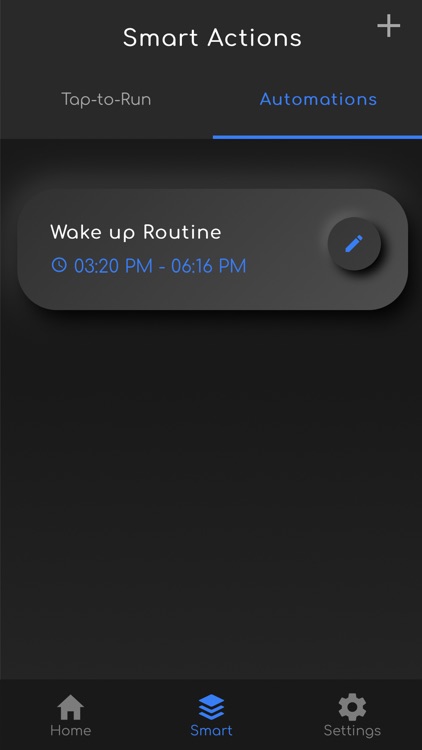The image displays a digital interface with a prominent black box at the top labeled "Smart Actions" in white text. To the right of this label is a grayish plus sign. On the left side of the box, it reads "Tap-to-Run," a directive presumably for user interactions, followed by the word "Automations" highlighted in blue underneath a thin blue line.

The main interface features a dark, almost black background with a foreground element in a grayish hue. Centered within this foreground is the label "Wake Up Routine" in white text. Beneath this label, there is a blue clock icon accompanied by the time range "03:20 PM - 06:16 PM." Next to this time display is a circular icon with a blue pencil in the middle, suggesting an edit function.

At the bottom of the screen, a light gray navigation bar includes several buttons. The leftmost button appears to be the home screen button. Adjacent to it is a blue button labeled "Smart." Following this is an icon of three diagonally stacked squares. Finally, on the far right of the navigation bar is a gray settings button, visually identified by an icon resembling a six-pointed gear or screw head.